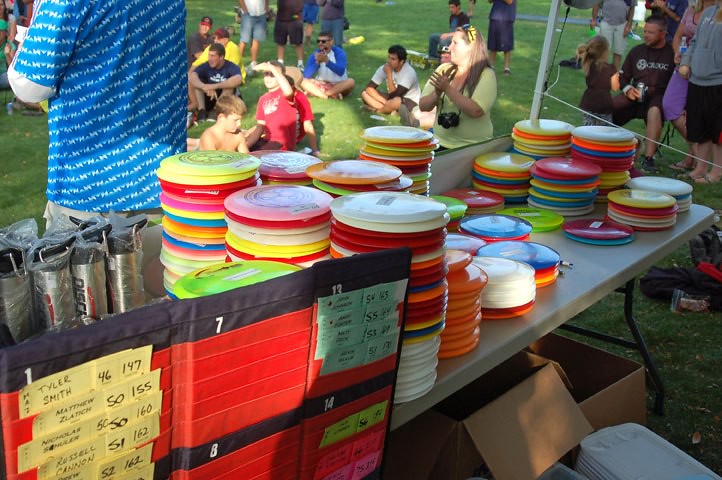This image captures a vibrant outdoor event, possibly a festival, children's track and field day, or company picnic, held during daytime. In the foreground, a long white table is stacked high with dozens of colorful frisbees in an array of colors including white, orange, blue, green, and yellow, each marked with logos. Nearby, some bins and coolers can be seen, filled with additional frisbees, water bottles wrapped in thin plastic bags, and other items. Beneath the table, cardboard boxes and a plastic bag are visible. To the left, bins are red and numbered, containing labels with people’s names and numbers. In the background, people of all ages sit on the bright green grass, some with their feet crossed, others in foldable chairs. Among them, a person in a blue shirt and shorts and another wearing a yellow shirt with a camera stand out. The scene exudes an air of community and fun, characterized by the colorful attire and lively atmosphere.